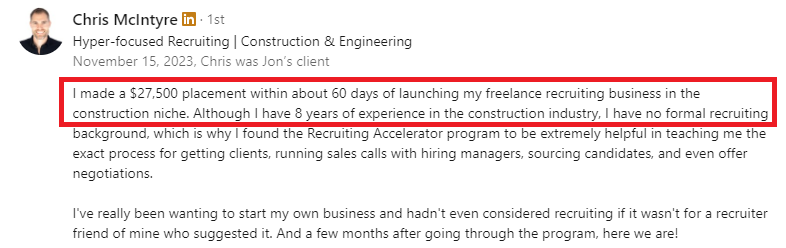This is a detailed screenshot with a white background. In the upper left-hand corner, there is a profile icon featuring a man's picture. To the right of the icon, the name "Chris McIntyre" is displayed in bold, gray text. Adjacent to the name, there is a brown box with the LinkedIn logo, which consists of the letters "IN" in white. Moving further right, there is a midline gray decimal point followed by the text "1ST" in gray.

Two lines below, in black text, it reads "Hyper-Focused Recruiting" followed by a vertical black line and then "Construction and Engineering." Below this line, in gray text, it indicates "November 15, 2023," along with the statement "Chris was John's client."

The content below this is divided into two paragraphs, with the first two lines prominently outlined with a thick red line. The highlighted text states: "I made a $27,500 placement within about 60 days of launching my freelance recruiting business in the construction niche. Although I have eight years of experience in the construction industry, I have no formal recruiting background." 

Following the highlighted section, the text continues: "which is why I found the Recruiting Accelerator program to be extremely helpful in teaching me the exact process for getting clients, running sales calls with hiring managers, sourcing candidates, and even offer negotiations."

The second paragraph begins: "I've been wanting to start my own business and hadn't even considered recruiting if it wasn't for a recruiter friend of mine who suggested it. And a few months after going through the program, here we are!"